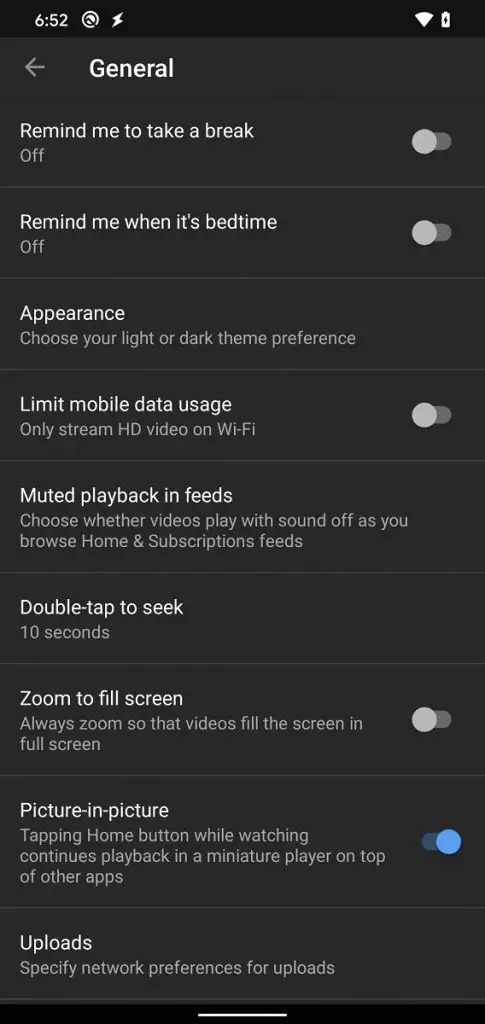This image is a screenshot taken from a cell phone, displaying a settings menu. The background is black with white text, typical of many modern user interfaces. In the upper left corner, the time is shown as 6:52, accompanied by various standard status indicators such as a lightning bolt symbol. On the right side, there are the battery and WiFi symbols, indicating the phone's connectivity and battery status.

Below the status bar is a gray header bar labeled "General." This section includes various toggle options that users can turn on and off. 

- The first option is "Remind me to take a break," which is currently turned off. The toggle button is gray and positioned to the left.
- The second option, "Remind me when it's bedtime," is similarly off, with its toggle button also gray and to the left.
- Following that is the "Appearance" section, where users can choose their light or dark theme preference—though no toggle button is shown here.
- The "Limit mobile data usage" option is next, followed by the "Only stream HD video on WiFi" setting, both of which are turned off.
- The "Muted playback in feeds" setting is listed next but does not indicate its current status.
- The "Double-tap to seek" feature is similarly mentioned without any visible toggle status.
- The "Zoom to fill screen" option, which ensures videos always fill the screen fully, is turned off, with its toggle button gray and to the left.
- The "Picture-in-picture" mode, which allows for miniaturized playback while multitasking, is enabled; its toggle button is blue and positioned to the right.
- Finally, at the bottom of the list, there is an "Uploads" section.

Each feature is separated by lines for clear demarcation, providing a visually organized and comprehensive settings menu.